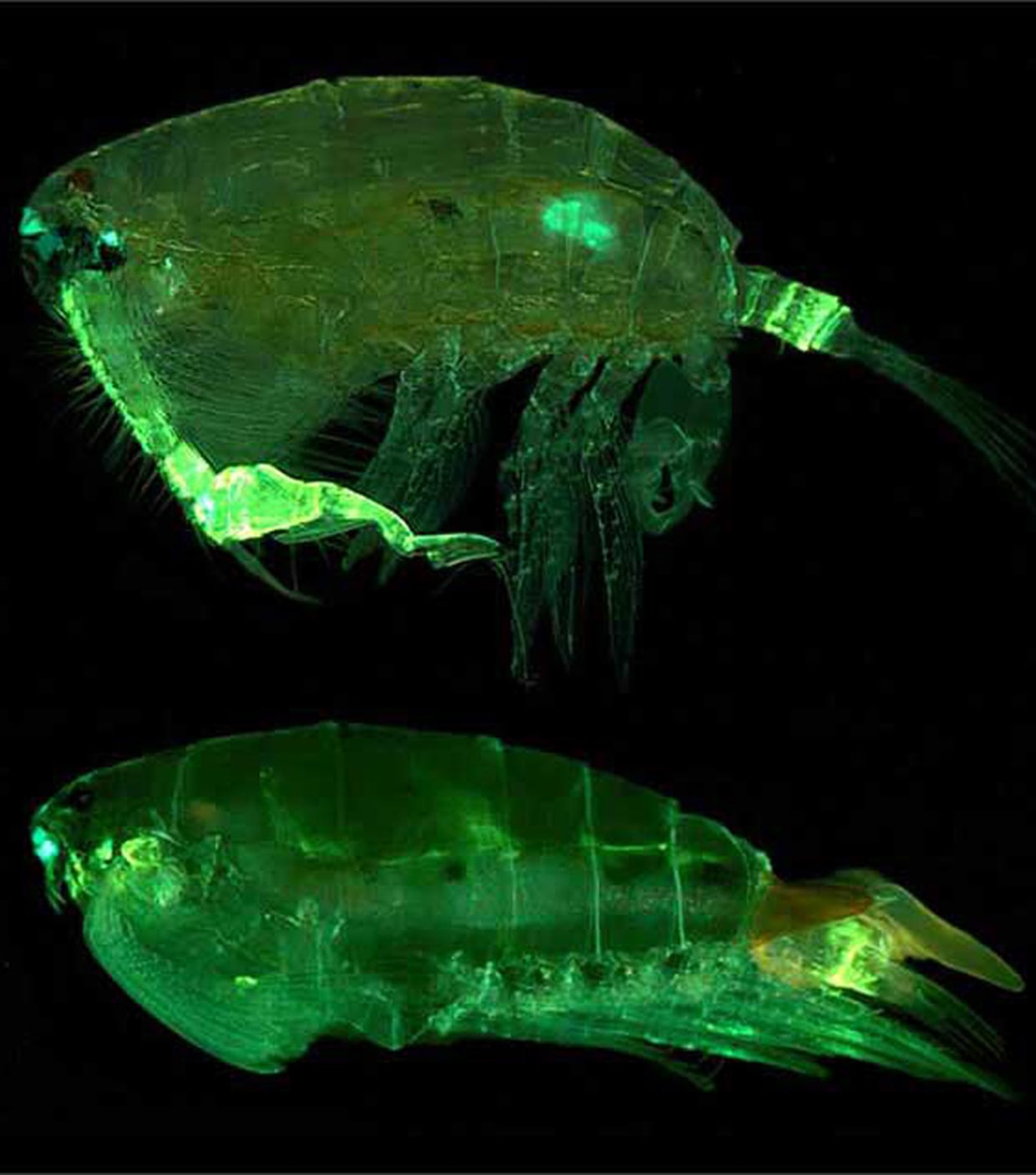This image captures two small, possibly microscopic sea creatures exhibiting phosphorescence against a stark black background. Each creature glows neon green while their translucent bodies suggest a bioluminescent quality that stands out vividly in the darkness. Both are oriented towards the left side of the image; their hard, shell-like upper bodies contrasting with the fin-like appendages underneath. The upper creature's leg fins are extended, giving a detailed view of their intricate structure, while the lower one's fins are tucked in, creating a streamlined shape. Notable bright green highlights are visible at specific points, such as the head and tail, showcasing the unique luminescent properties of these intriguing marine organisms.